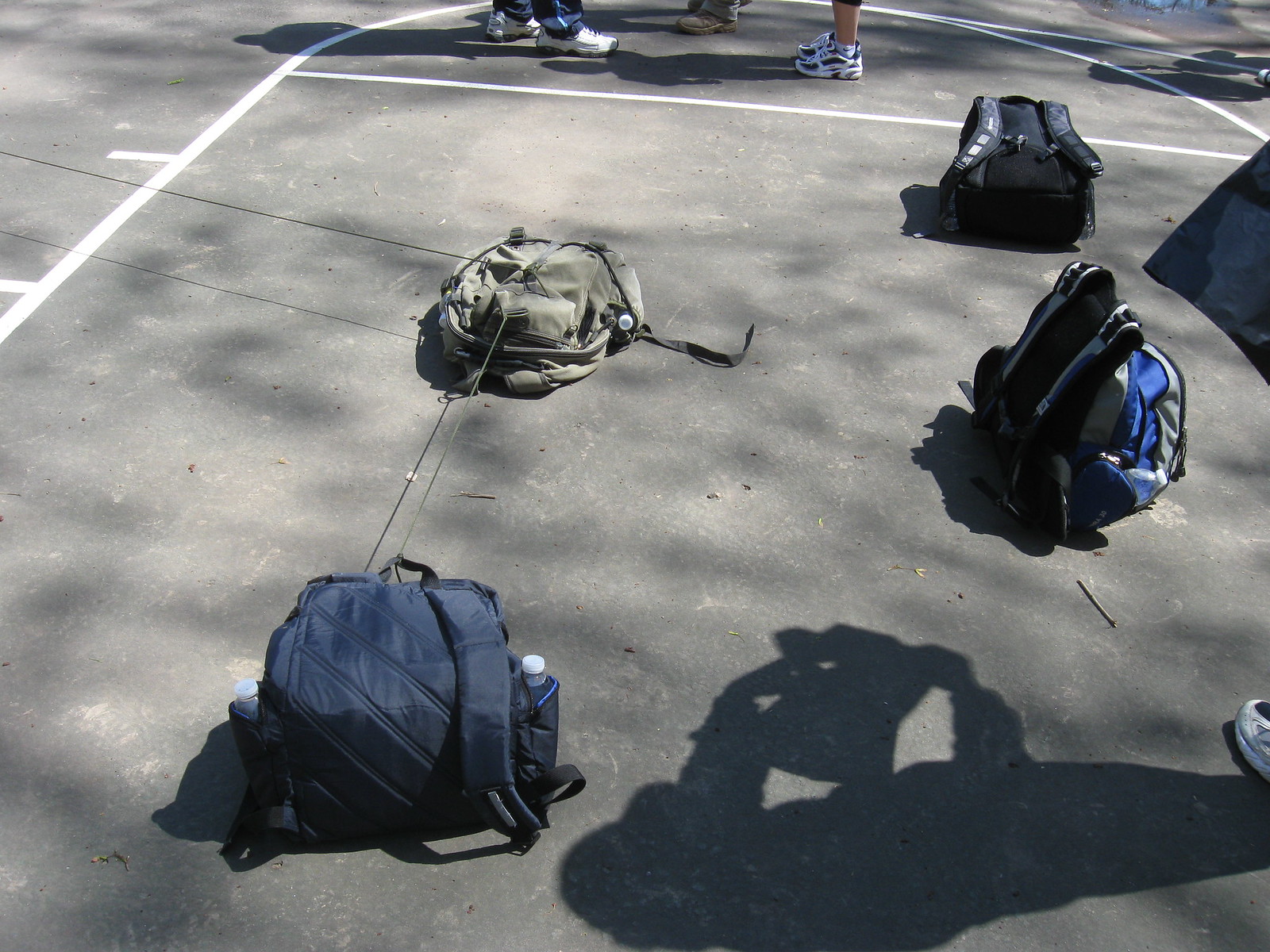The photograph showcases a section of an outdoor basketball court, specifically the key area with clearly visible three-point and foul shot lines. In the upper portion of the image, three individuals, likely students, stand with only their lower legs and sneakers visible. One of these individuals appears to be Caucasian, wearing shorts. The court's surface is littered with minor debris such as small twigs and dirt.

In the lower part of the image, four backpacks are arranged on the ground in a loose pattern, possibly indicative of placeholders. Closest to the viewer is a blue backpack, followed by an army green backpack with a water bottle in its pocket. Adjacent to it, a blue and black backpack is positioned on its side, exposing the straps, and finally, another large blue and black backpack lies flat on its front. A string stretches between two of the backpacks, forming an "L" shape. Notably, the shadow of the person taking the photo is visible in the bottom right, revealing they are using a tablet. Their foot also appears in the lower right corner, edging into the frame.